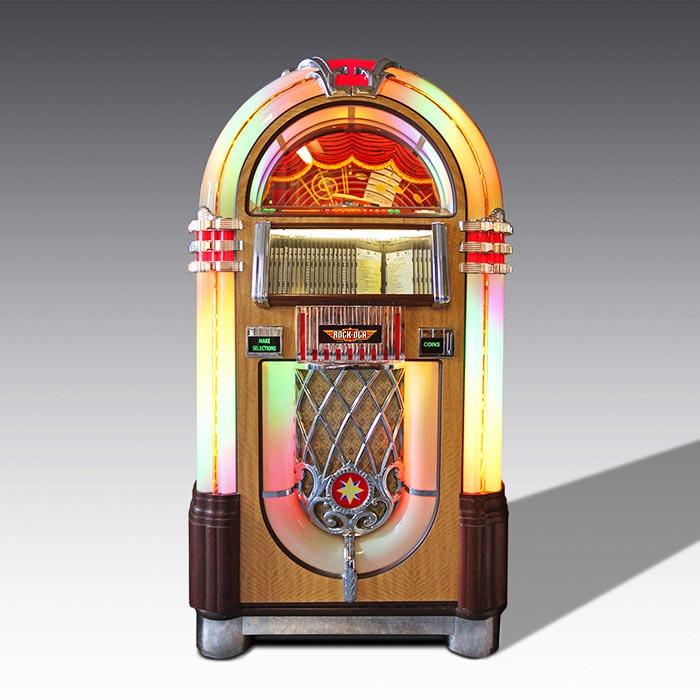On a grey background, there stands a beautifully detailed vintage jukebox with a rounded top. The jukebox features a prominent red section bordered by gleaming silver metal. Bright, colorful lights adorn its sides: orange and yellow hues at the top, followed by dual red strips separated by silver metal, and transitioning into yellow, orange, and pink at the bottom. The base of each side is accented with a black strip. It stands on sturdy silver metal legs. At the center, a clear window showcases an array of CDs to choose from, framed by a vibrant U-shaped design in green, yellow, pink, and orange. The jukebox also includes coin slots for operation, completing its classic look.